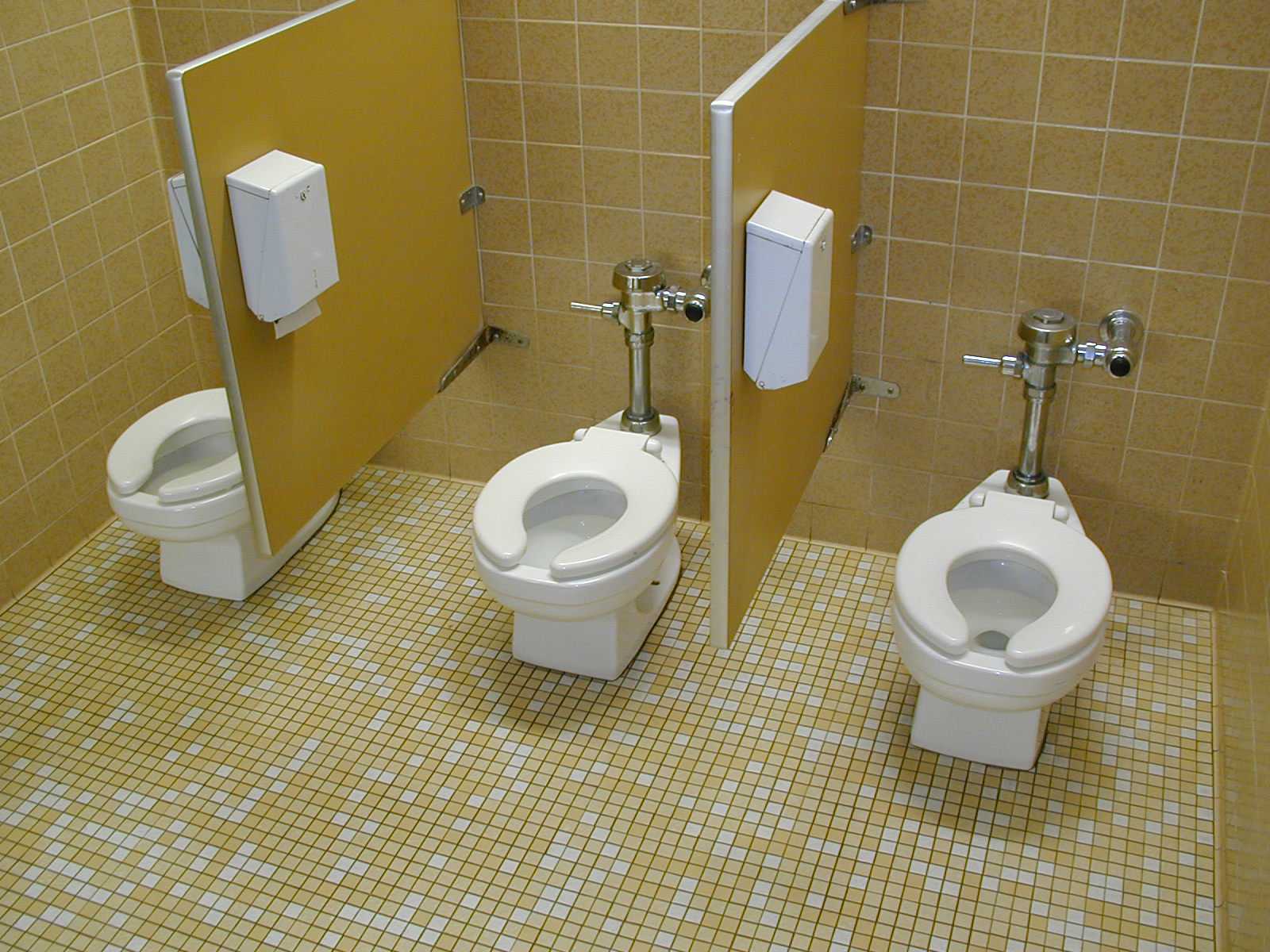This image captures the interior of a public restroom likely over 20 years old, characterized by its distinct tiling and layout. The floor is composed of very small, goldish and white tiles arranged in a mosaic pattern with grout in between. The walls feature larger golden brown tiles with white grout. There are three white toilets, all identical and child-sized, each positioned within a partitioned area without doors, offering no privacy. These partitions are a light-colored yellow-orange hue with silver edging. Each toilet has a silver tone pipe system for flushing and lacks a traditional tank or lid. Above each toilet is a white box dispenser that appears to provide paper, possibly in sheets rather than rolls, resembling a paper towel holder more than a conventional toilet paper dispenser.